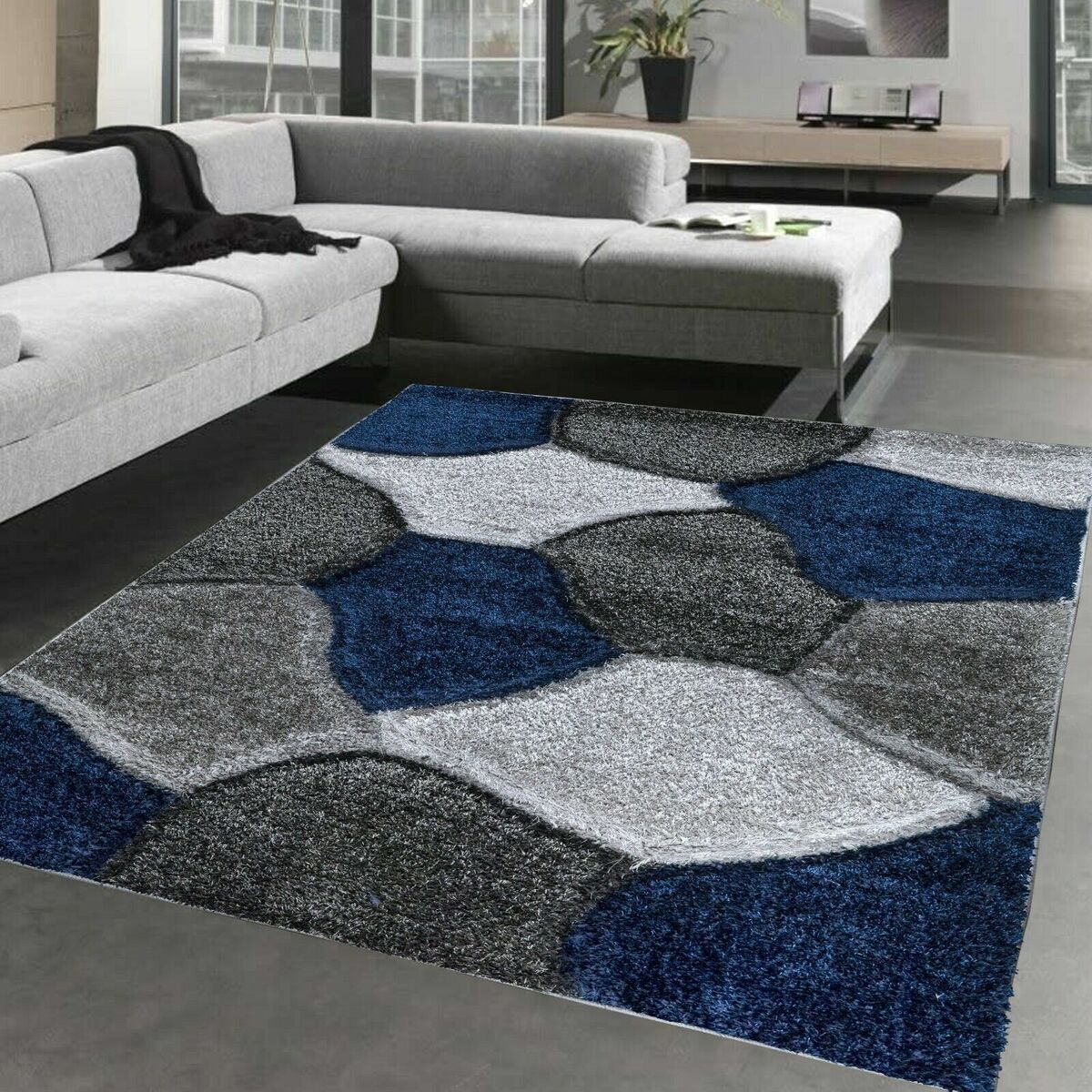This image showcases a professionally staged, modern living room, likely intended for a magazine or a website. The central piece is a large grey sectional couch arranged at a 90-degree angle, adorned with a black throw blanket and flanked by scattered magazines. The flooring is a sleek stone grey, covered partially by a vast, rectangular area mat featuring an abstract splotch design in blue, white, and grey, which adds vibrant color to the neutral tones of the space. 

Additional elements that enhance the room's aesthetic include a green plant in a black vase, a tan table, and a piece of artwork or possibly a mirror hanging on the neutral-colored walls. Natural light filters through the windows on both the left and right sides, illuminating the space and highlighting its contemporary style. Overall, this meticulously arranged living room encapsulates modern design with a blend of muted and vivid hues.